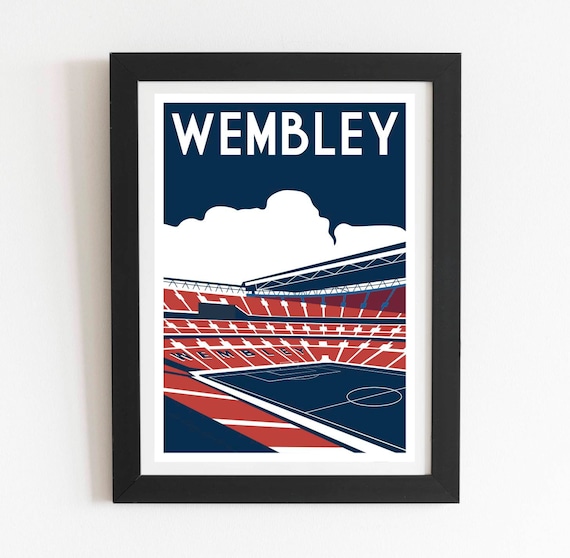A framed picture hangs on a light gray wall. The frame is black, encasing a light gray border followed by a smaller white border. The centerpiece is a detailed, colored drawing capturing a panoramic view of Wembley Stadium. At the top of the image, large white letters boldly spell out "Wembley" against a blue sky, dotted with puffy white clouds. The stadium dominates the scene with its distinctive red seats and white aisles, creating a cohesive and vibrant visual. Diagonally across the image, blue rafters arc from just left of center to the right. The stadium field, depicted in blue, includes white markings: a central circle, the outlined goal, and a white horizontal line traversing the pitch. The scene is enhanced by the visible red bleachers on the lower left, and a blue triangle in the bottom left corner, possibly an awning. This artistic rendition encapsulates the grandeur and iconic elements of Wembley Stadium, emphasizing its importance and scale.